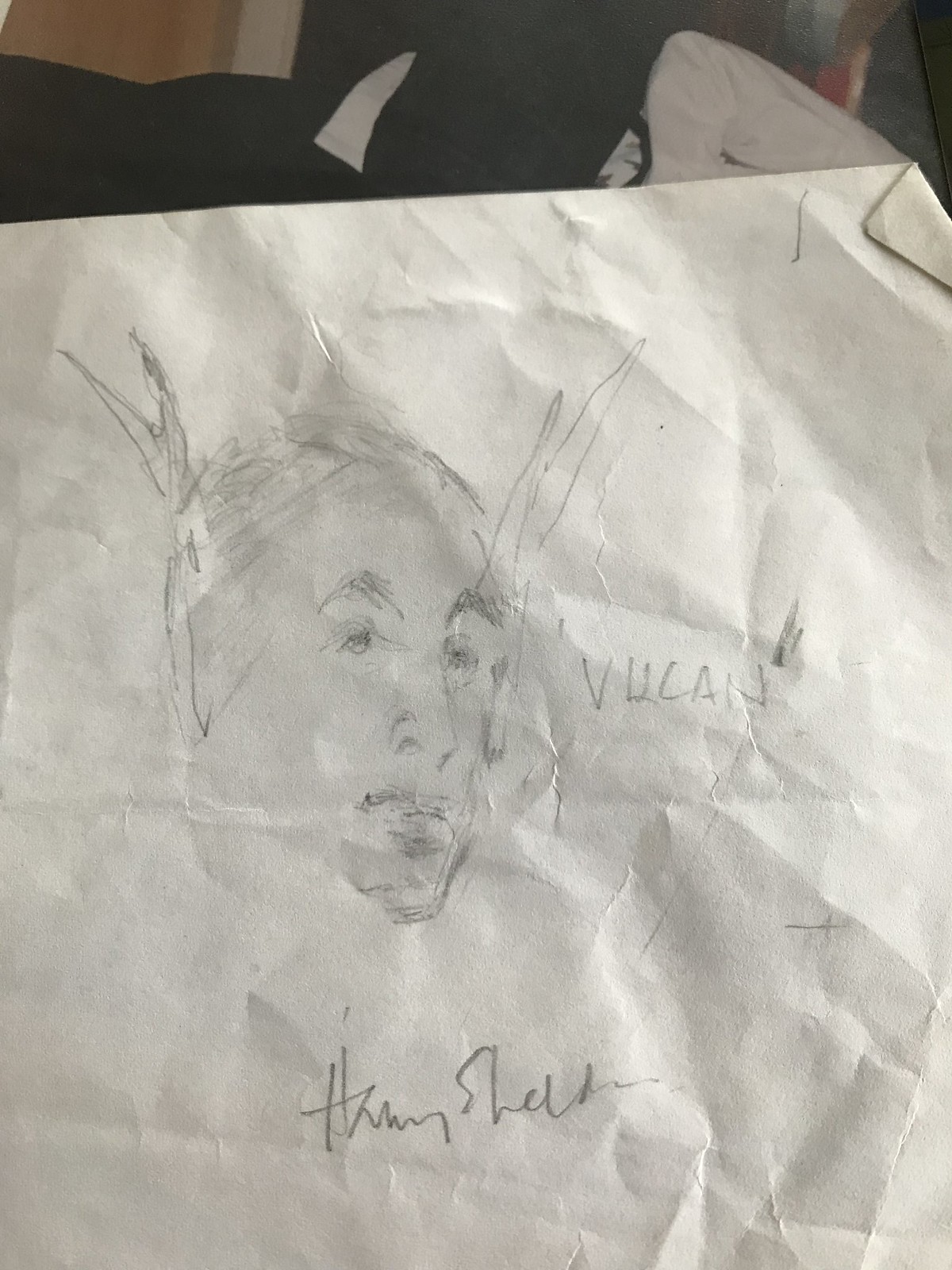A creased and slightly wrinkled piece of white paper lies unfolded, revealing a pencil sketch and a signature at the bottom. The upper right-hand corner of the sheet is subtly folded over. The sketch portrays a face with its head tilted slightly to the viewer's right. The figure has minimal hair, with what appears to be two horn-like objects emerging from the top of the head, though their exact nature is ambiguous. Dark eyebrows accentuate the eyes, which gaze off into the distance, and the face is framed by a straight nose and full lips, suggesting expressiveness. A glimpse of an ear and a partial chin completes the visage, next to which the inscription "V-U-C-A-N" is written. The cursive signature at the bottom is difficult to decipher but might read "Harry Sheldon." In the background, a neatly made bed with a black comforter and a white pillow is visible.